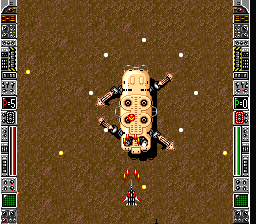This image is a screenshot from a video game, featuring a high-tech interface framing the scene on both the left and right sides. These frames are adorned with grey metallic graphics, intricate with various small numbers, letters, and dots that evoke a futuristic control panel. Dominating the center of the screen is a textured brown background with a dirt-like appearance, providing an earthy contrast to the technological elements.

At the bottom of the image is the player's avatar, a sleek red spaceship emitting four red bullets aimed upwards. The target of this assault is a tan robotic creature, positioned in the middle of the image. The robotic entity, resembling an insect, is segmented and supported by four limbs which give it a dynamic and slightly menacing posture. Suspended across the screen are scattered projectiles: white bullets clustering near the robotic creature, suggesting intense close-quarter combat, and yellow bullets further away, hinting at a broader range of conflict. The scene is a vivid snapshot of an intense intergalactic battle.